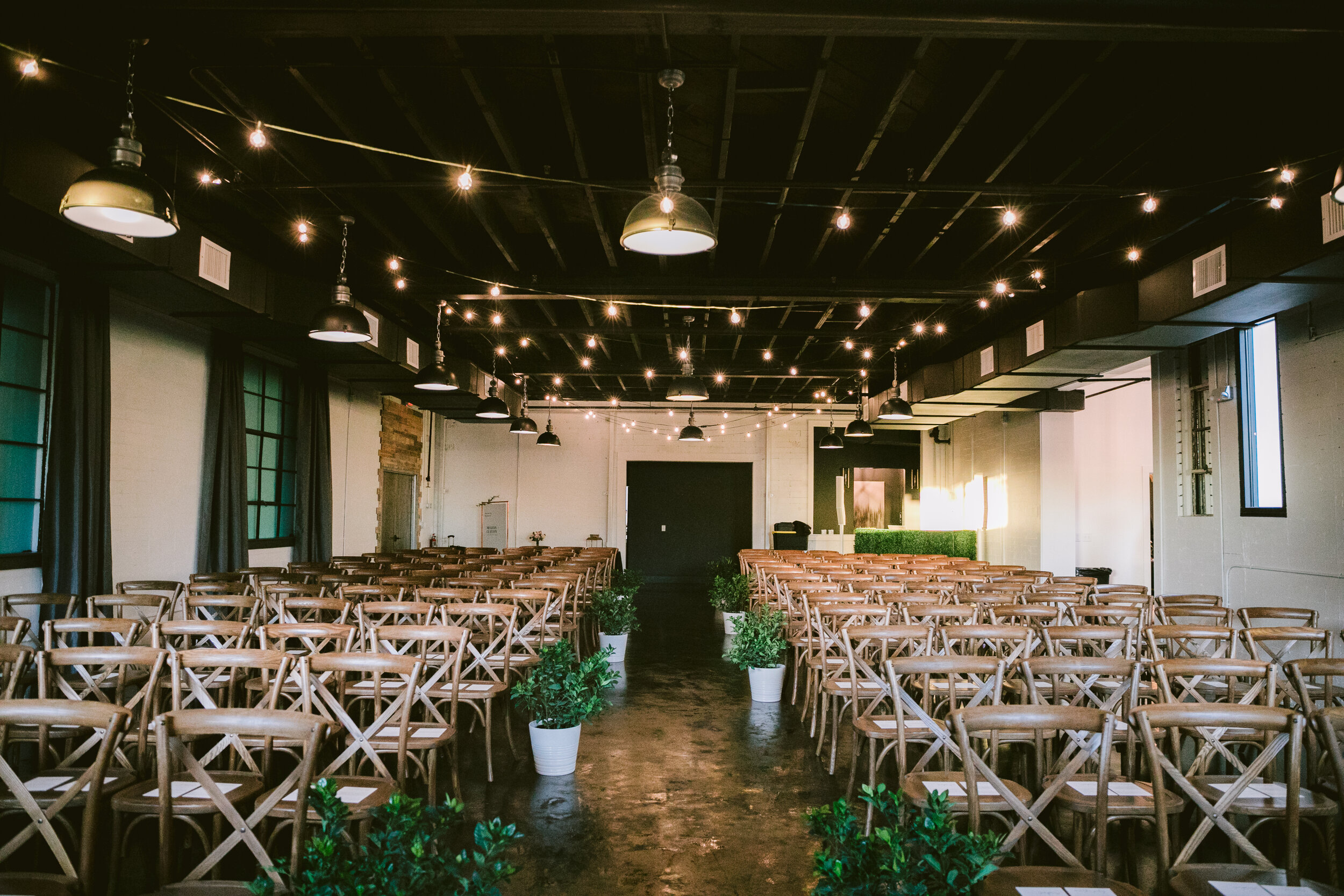This image depicts a beautifully prepared event space, potentially set up for a wedding or a formal gathering. The room features a high, dark brown rafter ceiling adorned with strings of delicate lights stretching zigzag across the length of the room, creating a cozy and inviting atmosphere. The floors are a dark bronze-gold stained concrete, enhancing the room’s elegance. Along each side of the central aisle, there are numerous dark brown wooden chairs with crossbacks, arranged in neat rows—approximately 25 in total. Each row is lined with white pots containing vibrant green plants, adding a natural touch to the decor. The off-white walls are complemented by large industrial-style windows, dressed with dark brown or gray curtains. At the front of the room, additional plants peak into view, reinforcing the room’s symmetrical and meticulously arranged setup.